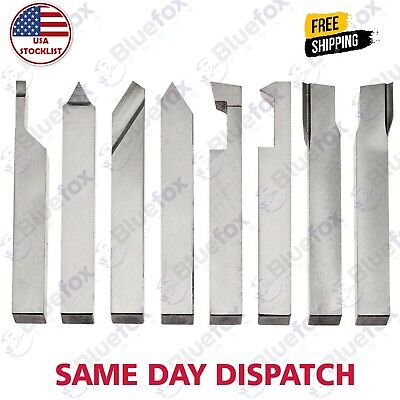This color photograph features eight metal tools, possibly carbide tips for lathes, that are neatly arranged in a horizontal row. Each tool is a thin, rectangular bar made of shiny silver metal with variously shaped cutting edges at the tips; some are pointed, some have sections cut out, while others resemble drill tips. Dominating the top left corner of the image, there's a circular emblem with the American flag and the words "USA Stock List" in bold red text beneath it. To the immediate right, a yellow and black label declares "Free Shipping." The bottom of the image is marked with red block text stating "Same Day Dispatch." A watermark with the text "Blue Fox" is repetitively overlaid across the entire photograph, indicating the brand.